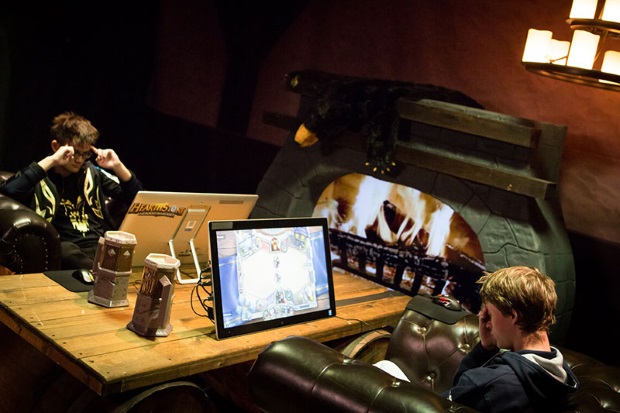The image depicts two young men, likely in their 20s or 30s, engrossed in a game of Hearthstone at a large wooden table designed to resemble an old pub. Each man sits in a large brown leather chair, facing dual monitors with built-in kickstands that display the game. Both players appear frustrated: the young man on the right, wearing a dark blue hoodie, has his palm over his head, showing his dirty blond hair, while the man on the left, dressed in a black t-shirt, points two fingers from each hand towards his temple. He sports short brown hair and glasses. Their setup includes octagon-shaped beer steins with a medieval, pixelated design. Behind them, a rustic fireplace featuring a bearskin rug draped over a stone mantle adds to the ambiance, while an LCD screen within the fireplace simulates a roaring blaze. A lighting fixture with faux candles hangs in the top right corner, completing the cozy, historical atmosphere. Two mugs are also neatly placed on either side of the desk, contributing to the scene's intricate detailing.